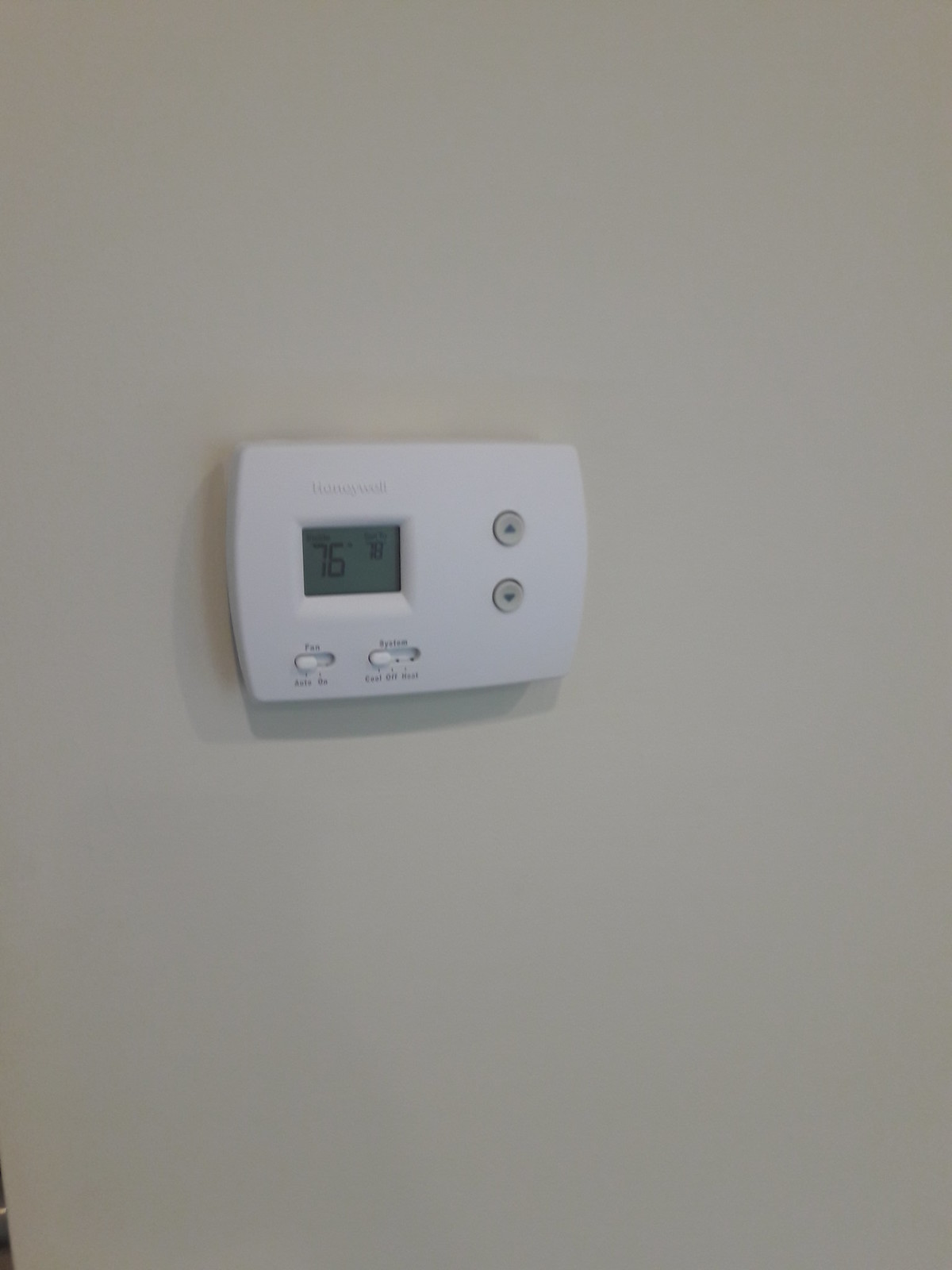A sleek, white Honeywell thermostat is mounted on a cream-colored, off-white eggshell wall. The thermostat, rectangular in shape, features a clear digital display indicating the current room temperature is 76°F, while the set temperature is 78°F. The system mode is set to 'Cool,' and the fan is on 'Auto,' suggesting the central air will activate as needed to maintain the desired temperature. The thermostat includes subtle, white-on-white embossed branding that reads "Honeywell." Below the display, two transparent arrow buttons—one pointing up and one pointing down—allow for easy temperature adjustment.